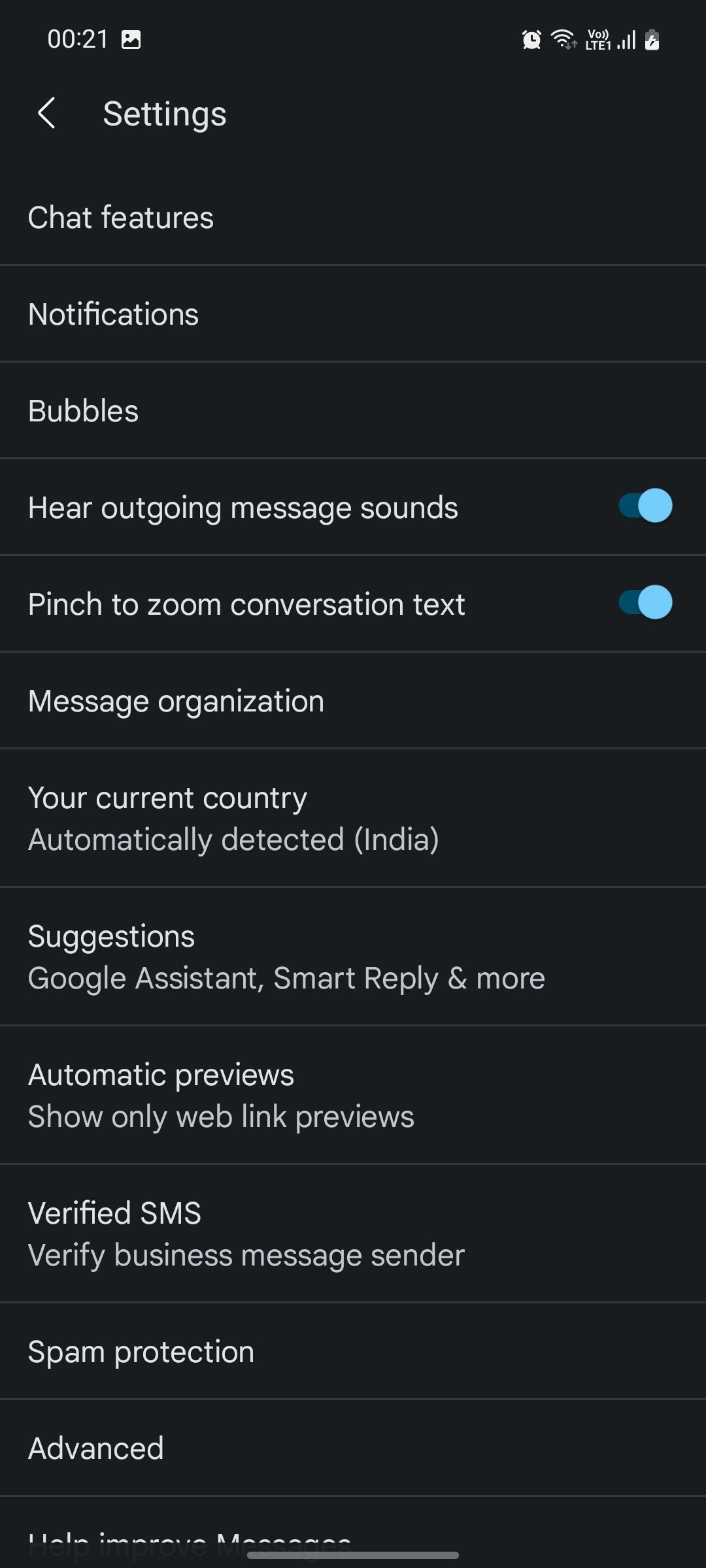The image portrays a black screen in a phone format, characterized by its long and tall dimensions. At the top left corner, "00:21" indicates the time, accompanied by a picture icon. The top right corner displays indicators for "VOD LTE," battery status, Wi-Fi connectivity, and an alarm icon.

On the left side, the screen label "Settings" is written in white, paired with a left-pointing arrow. Below this, various menu options are listed, each separated by a line. These options include:

1. Chat Features
2. Notifications
3. Bubbles
4. Hear Outgoing Message Sounds (showing a blue toggle switch activated)
5. Pinch to Zoom Conversation Text (also with a blue toggle switch activated)

Following these are additional settings options, including:

6. Message Organization
7. Your Current Country: Automatically Detected India
8. Suggestions
9. Google Assistant
10. Smart Reply and More
11. Automatic Previews
12. Show Only Web Link Previews
13. Verify SMS
14. Verify Business Message Sender
15. Spam Protection
16. Advanced

At the bottom, partially visible text hints at options related to Help and Messages, but the content is cut off and not fully legible.

Overall, the screen captures a comprehensive view of message settings and options available on a mobile device.